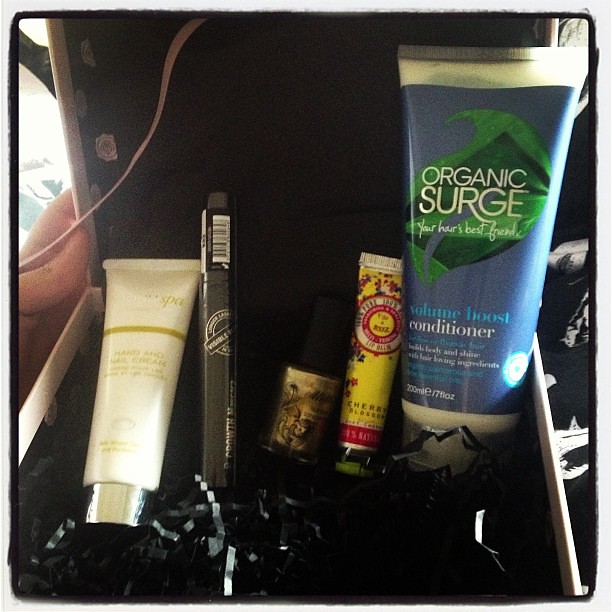The image captures a detailed close-up of an open black interior box, likely a gift set, showcasing a variety of cosmetic products arranged neatly. At the base of the box, black shredded paper mimics Easter basket grass, providing a backdrop for the products that are propped up against the back lid. The first item on the left is a white tube, elaborately designed with gold accents and unreadable gold text. Next, there is a cylindrical, cigar-shaped black object with a gold stripe and a barcode at the top, possibly a makeup stick. The third item appears to be a small light brown bottle, barely visible with a black cap, indicating it is likely nail polish. Adjacent to this is a yellow tube with red and white text, identified as cherry blossom lip balm. The largest item on the far right is a blue tube labeled "Organic Surge" in white font, featuring a green leaf logo and described as a conditioner. Completing the scene, a person’s left hand holds the box open, highlighting the juncture between the lid and the main compartment. The box lid is also accented with a white rim, and outside the box on the left, a ribbon and a hint of pink detail are visible, adding to the ornate presentation.